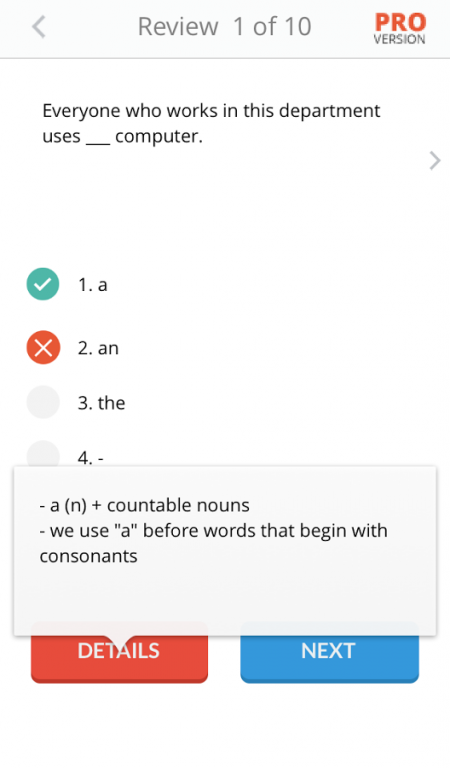**Detailed Caption for Image:**

The image is a screenshot of what appears to be a software interface, with a white background. At the very top center, the text "Review 1 of 10" is displayed in gray font. In the upper right corner, the word "PRO" is written in bold red capital letters, with "VERSION" directly below it in smaller gray capital letters. On the left side, an arrow points to the left, followed by a thin vertical line that separates this section from the rest of the page.

Below this line, the text "everyone who works in this department uses" appears in gray font, with a blank line (underscore) indicating a missing word. A small arrow is visible at the far right. This line is part of a fill-in-the-blank test where the user must choose the correct word.

Four answer options are provided:

1. The correct answer, "a computer," is marked as option A and is highlighted by a green circle with a white checkmark.
2. Option B, "an," is incorrect and is marked by a red circle with an X.
3. Option C, "the," is also incorrect.
4. Option D is hidden by a pop-up box.

The pop-up box is outlined in gray and contains detailed information about countable nouns. It features the text: "A (N) + countable nouns" followed by "We use 'A' before words that begin with consonants."

The pop-up box partially obstructs two rectangular buttons at the bottom of the interface. The left button is red and labeled "details," while the right button is blue with the word "next" in white lettering.

Overall, the screenshot illustrates a part of a language instruction or assessment tool, focusing on the correct usage of articles before countable nouns.